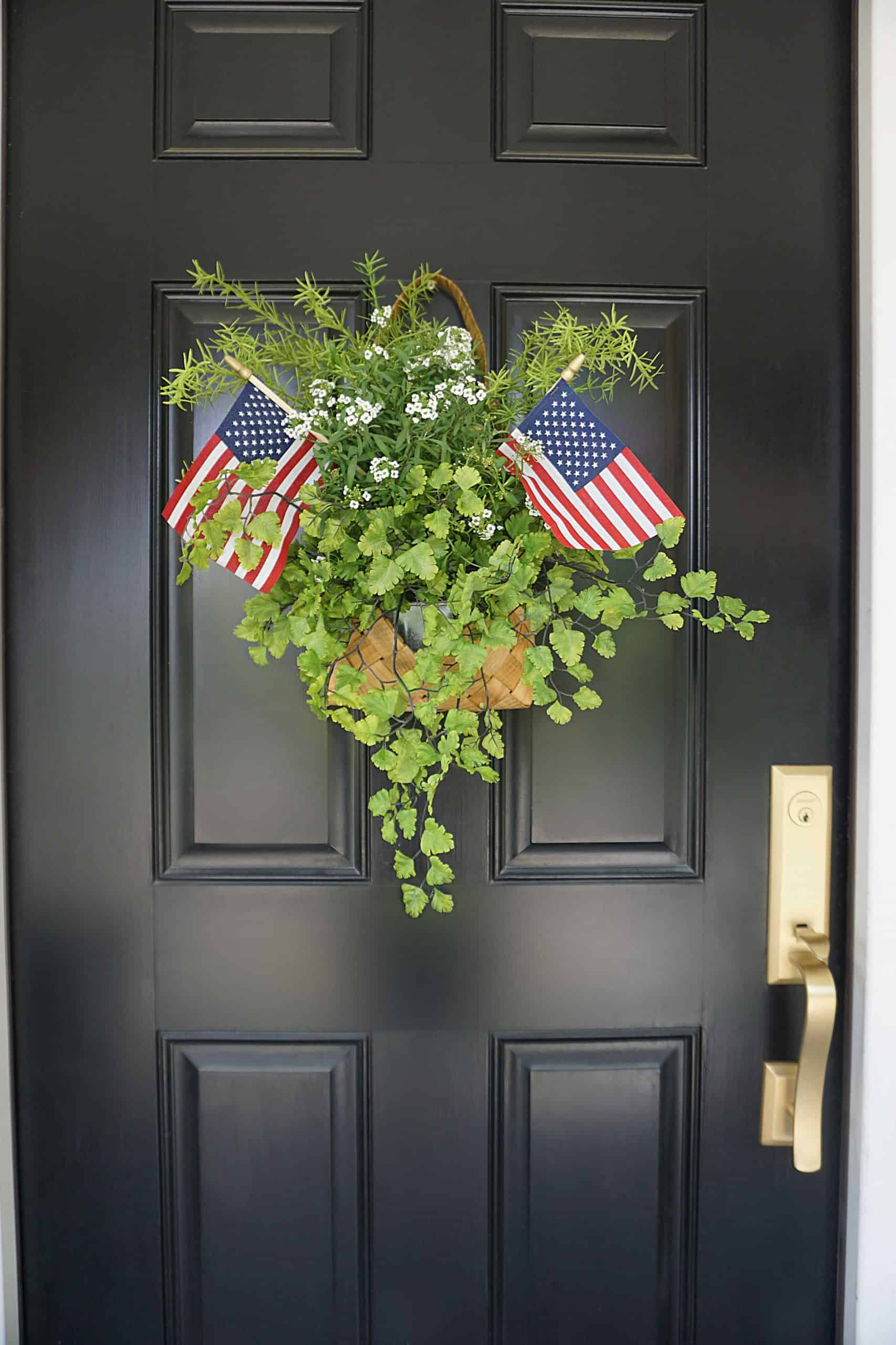This image captures a black wooden front door adorned with intricate architectural details. The door features six tall, vertically-oriented rectangular panels. Centered in the middle section hangs a woven wicker basket, brimming with lush green vine plants. Nestled among the foliage are delicate white baby's breath flowers, providing a soft contrast to the greenery. Additionally, two small American flags are prominently positioned on either side of the basket, adding a patriotic touch. The door is equipped with a gold handle, latch, and a centrally-placed keyhole, all of which stand out against the dark surface. The scene is framed by a white surrounding wall, highlighting the door's elegant yet welcoming design.